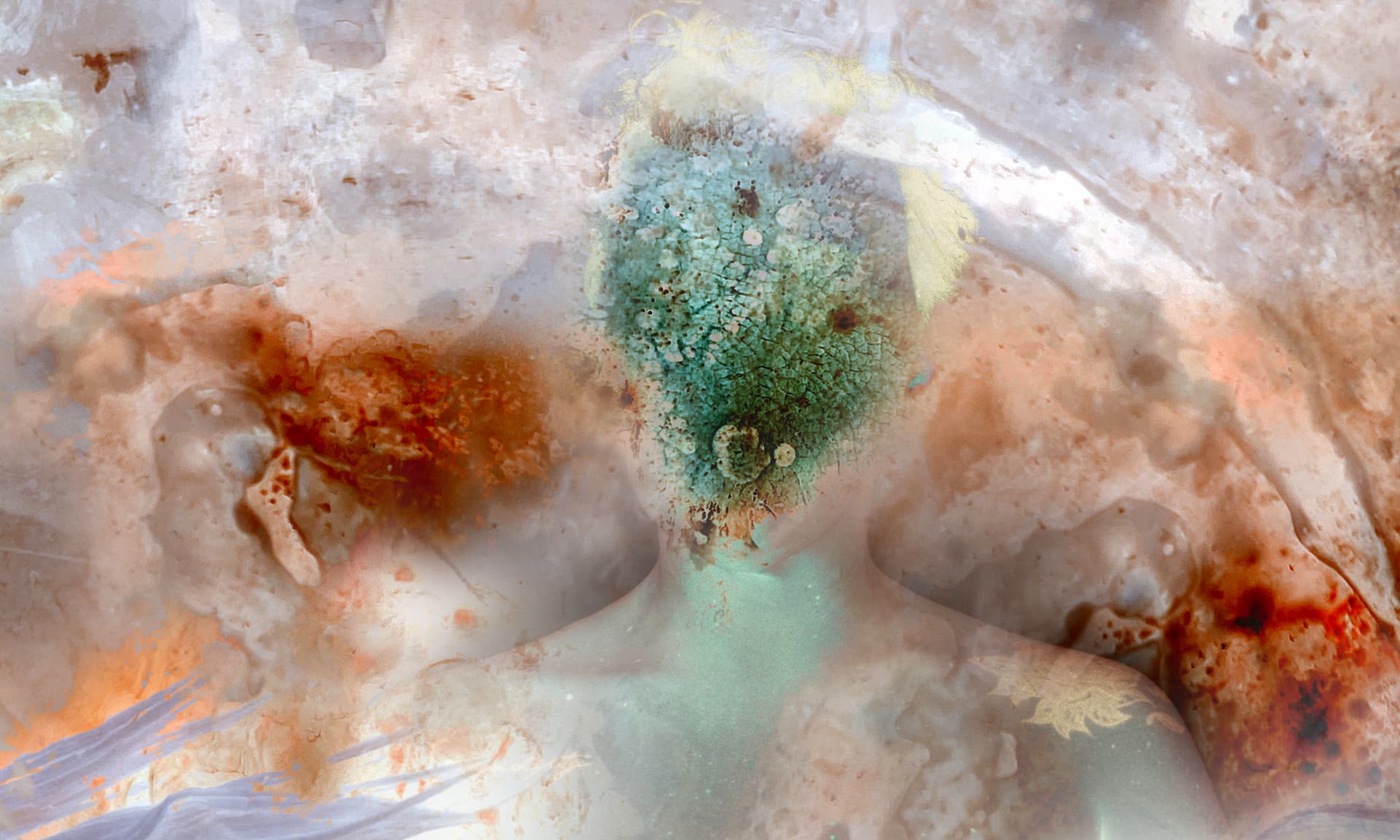This image presents a complex and abstract scene, reminiscent of a modern art collage, viewed from above without any specific borders. The background is a slushy, creamy white with shades of gray and beige, slightly tinged with brown. Dominating the center of the image, there is a large, green, somewhat diamond-shaped section mixed with light and dark green hues, and dotted with darker circles within it. This central green area seems to bleed color downwards, adding a subtle dynamic effect.

On the right side, a prominent, irregularly shaped brown blob is visible, featuring a lighter beige protrusion. To its right, there is an oblong-shaped blob that starts with a beige tone, similar to the background, but transitions into a reddish end. Both these shapes bleed their colors outward, adding to the layered and textured appearance.

Additionally, there's a noticeable darker section in the bottom-left corner, with colors ranging from dark red to almost black. Another similar, though distinct, darker area resides slightly off-center to the left, contributing to the image's intricate and enigmatic composition. The overall palette includes subtle hints of orange, blue, black, and red, enhancing the multifaceted visual experience. The interplay of colors and shapes creates an artistic and intriguing tableau that defies simple categorization.